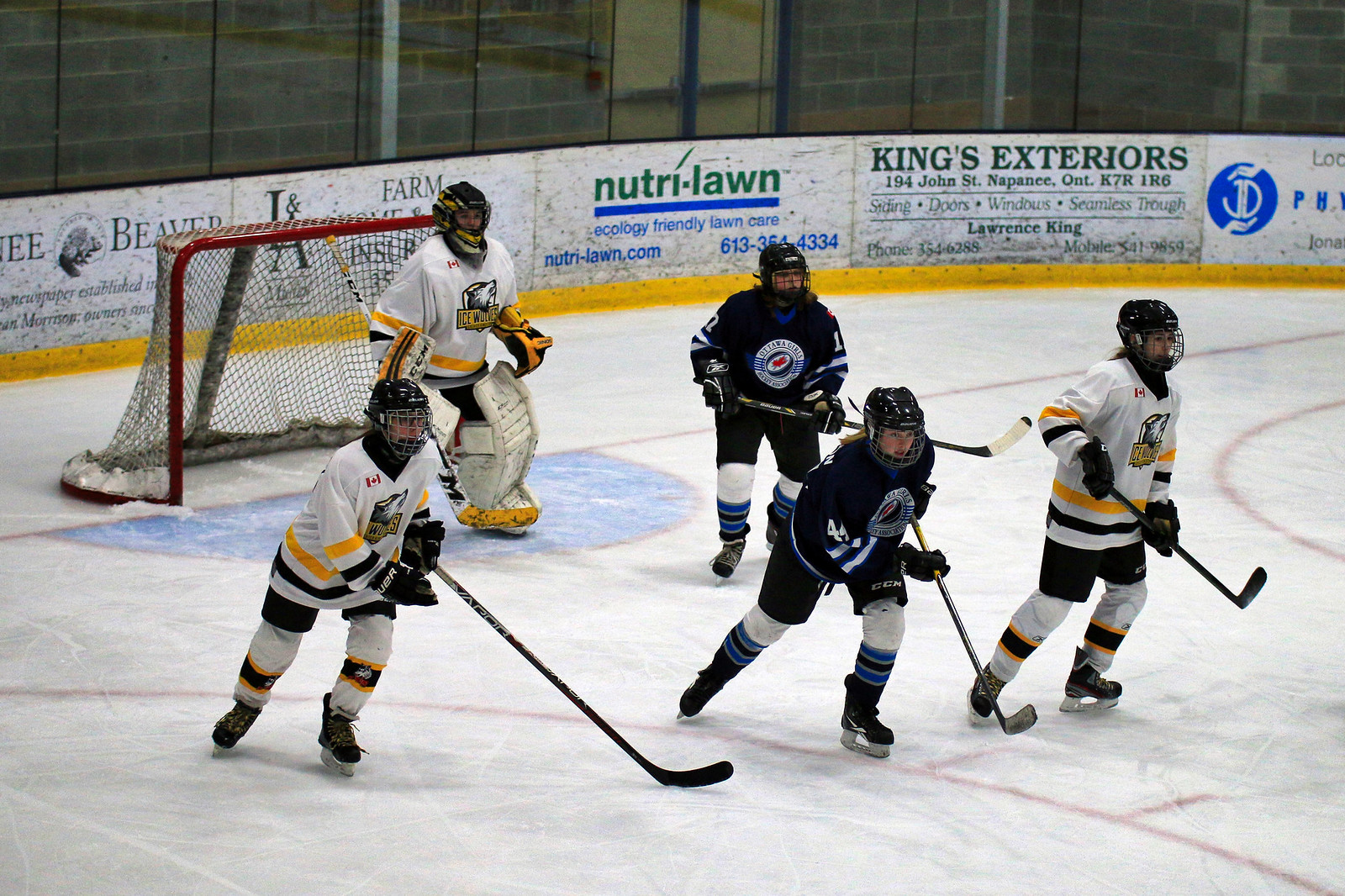In the image, we see a practice ice hockey game featuring two teams on a rink with the typical circle and line markings. The left side of the photo showcases five players in action near a goal marked by a semi-circle. The white team's jerseys are accentuated with yellow and black stripes, while the black team's uniforms include distinct black shorts. Both teams sport black skates and wield black hockey sticks. A goalie stands alert in the goal area, and the surrounding ads on the rink's barrier - including those for King's Exteriors, Nutri-Lawn, Farm Insurance, and one partially visible with “...e” – are consistent elements of a typical hockey setting. Behind the players, a black screen and empty bleachers indicate a practice session. Above the rink barriers, glass panels reveal a view of a brick wall and exit doors. The players, seemingly an all-girls team, are poised and focusing on an incoming puck, ready to engage.